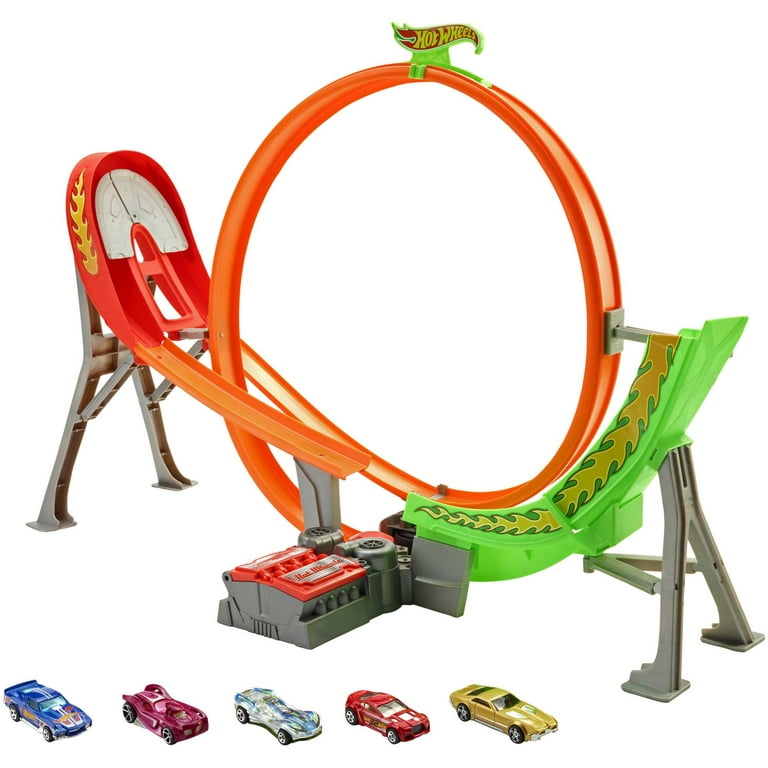This detailed photograph showcases a vividly colored Hot Wheels racetrack set on a white background. The track prominently features an intricate design, starting with a steep neon green ramp that leads into a vertically-oriented orange loop, complete with a full circle that curves back around into a red and green ramp descending further. The track is supported by a gray stand at the back and has gray legs holding up its sections. At the top of the track, the iconic "Hot Wheels" logo is clearly visible. Below the racing circuit are five toy cars, numerically detailed as a bright blue sports car, a burgundy muscle car, a white and blue-green custom car, a red vehicle, and a yellow model, all carefully arranged diagonally in the foreground.